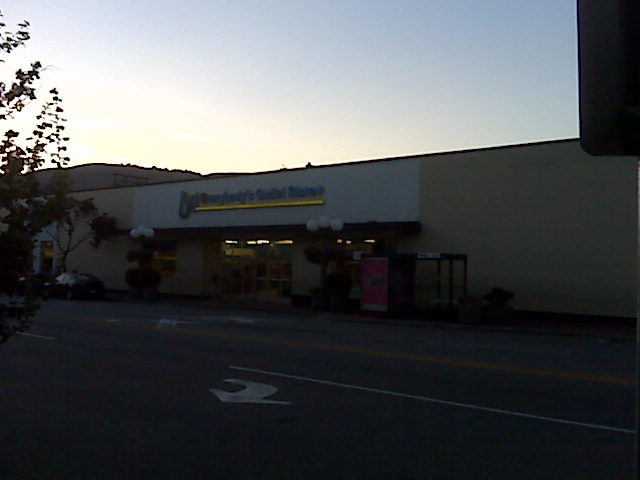In this image, we see a storefront taken from the perspective of a parking lot, with a road running alongside it marked with right-turn arrow signs. The store’s name, though difficult to decipher due to low lighting, is displayed in blue letters underlined by a yellow strip, set against a whitish background. The building itself is a grayish-beige color, though shadows obscure its exact hue. The sky, faintly blue, suggests it is either shortly after dawn or just before dusk, with light emanating from the left side of the image. A hill or mountain looms distantly above the store, adding depth to the background. In front of the store, there are unlit street lamps, a bus stop, and possibly tables or yard decorations. On the left, a tree and half a bush are visible. A street sign or parking lot sign is tucked in the top right corner. Finally, cars and a speed bump appear in the foreground, completing the scene filled with quiet, early morning or twilight ambiance.